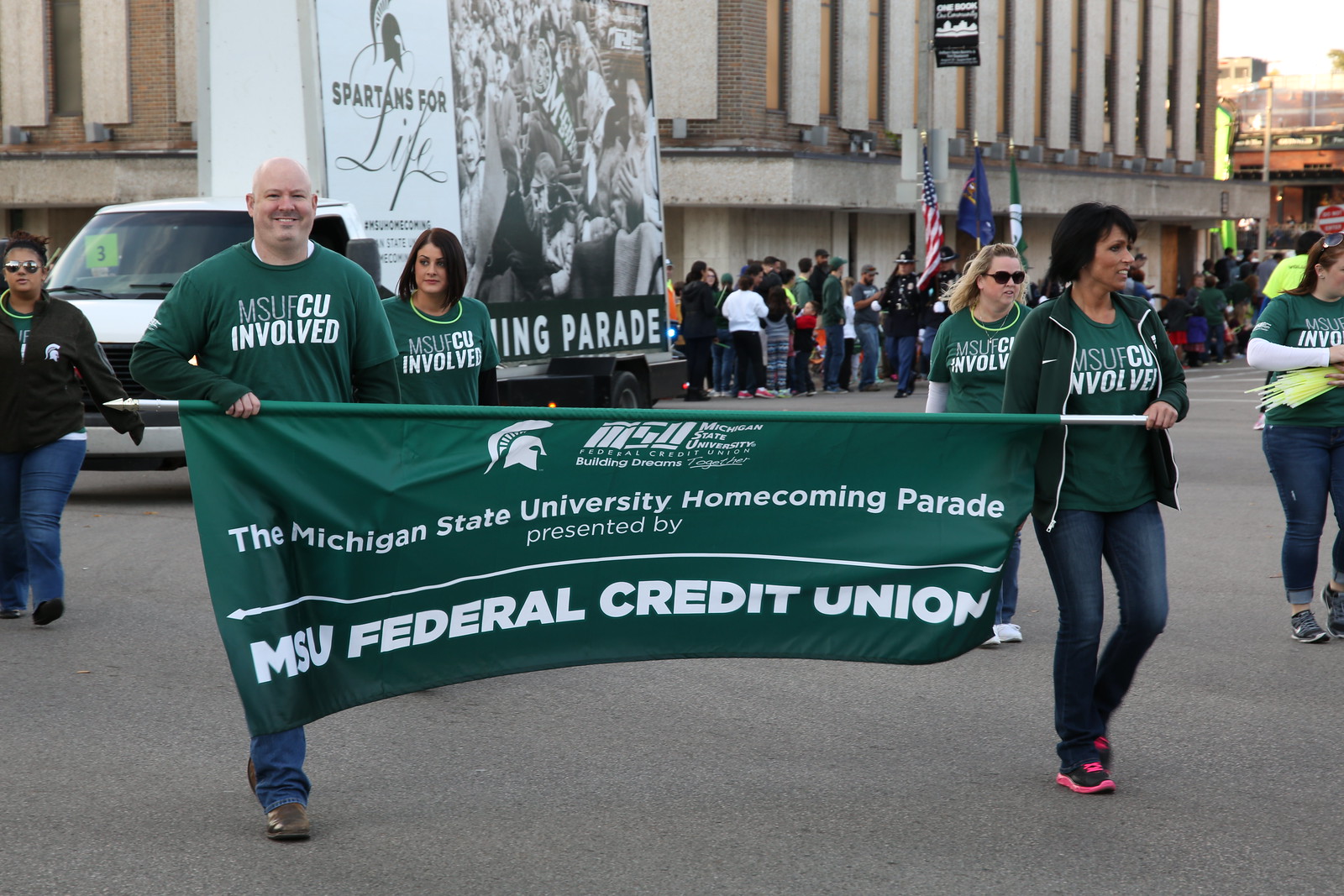In this image of the Michigan State University Homecoming Parade, a group of five individuals dressed in matching dark green MSU Federal Credit Union t-shirts and coordinating jackets are prominently featured. They carry a large, green banner with white lettering that reads "MSU Federal Credit Union Involved," further inscribed with "Michigan State University Homecoming Parade presented by MSU Federal Credit Union." A man on the left of the banner is sporting his green shirt over a black long-sleeve shirt, while the woman on the right also wears the same t-shirt with a green jacket and blue jeans. Behind them, a van follows closely, displaying a large sign with the phrase "Spartans for Life" and overseeing the parade's progress. Numerous spectators line the gray-paved street, many adorned in hoodies, jeans, and tennis shoes to stave off the chilly morning air. The scene is vibrant with American and MSU flags in the background, and one woman enthusiastically distributes glow-in-the-dark sticks from a large stack, contributing to the festive atmosphere as smiling participants and onlookers enjoy the parade.